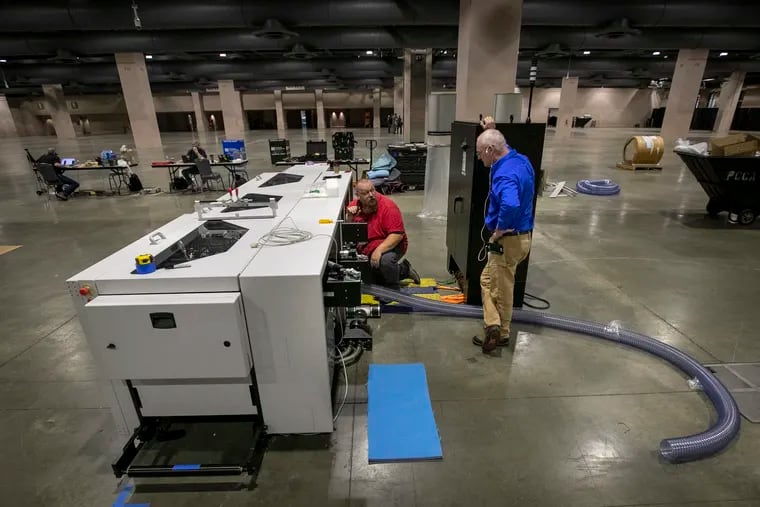The image depicts a vast, mostly empty indoor venue resembling an underground parking garage or large warehouse, characterized by concrete floors and pillars extending to a black ceiling adorned with small white lines. The focal point features an expansive white rectangular industrial machine situated at the front of the picture, with its right side connected to a long, clear plastic tube. Two men are engaged in examining the machine: one is kneeling in a red T-shirt, closely inspecting it, while the other, dressed in business attire with khaki pants and a blue shirt, stands beside him, leaning against a black file cabinet, hand on hip, and conversing with him. In the middle left area of the image, three long tables are positioned, with two of them occupied by single men. A garbage can is visible to the right, and in the background, a dumpster is overflowing with cardboard, adding to the scene's industrial and functional ambiance.